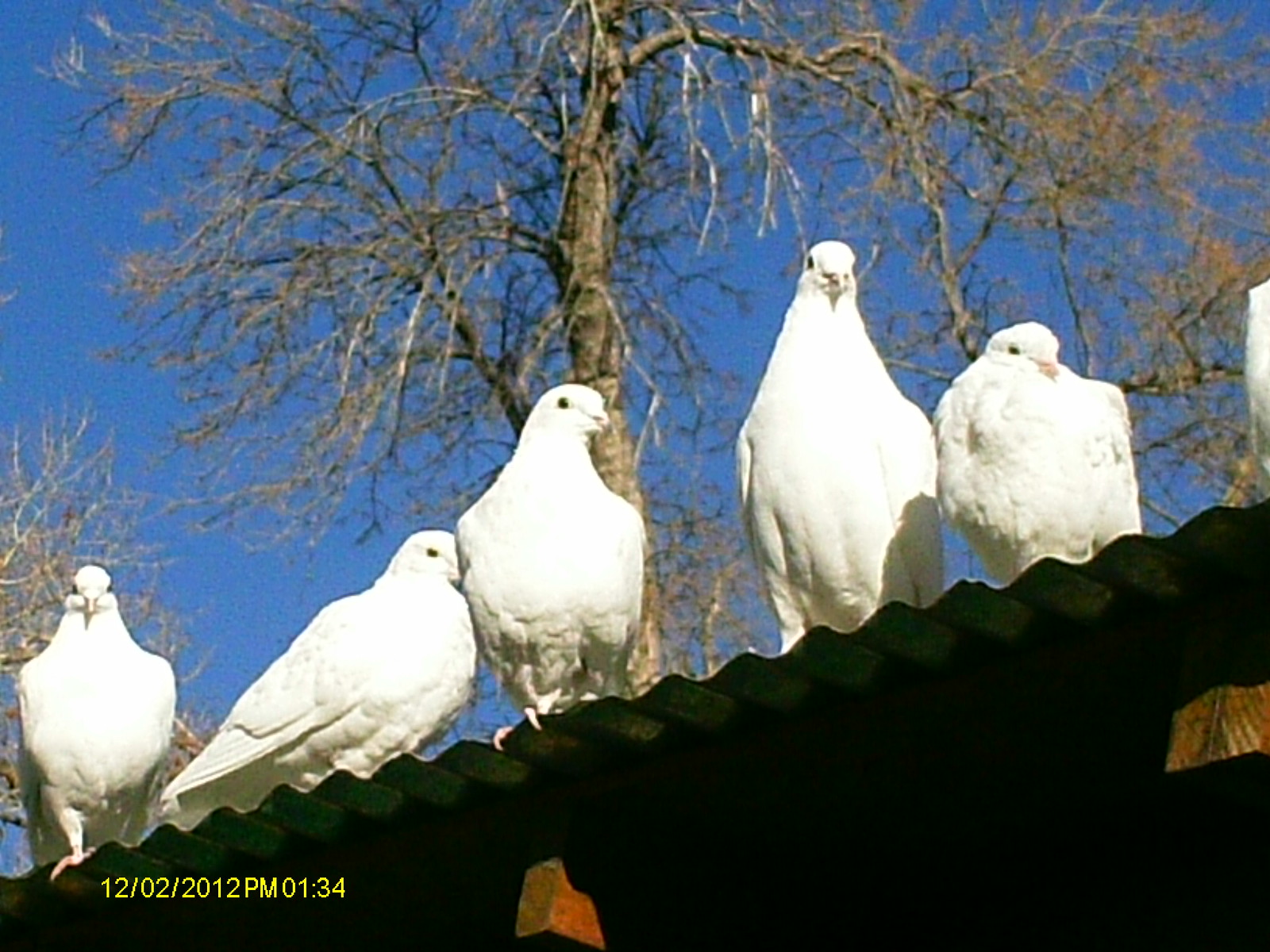This photograph, likely taken with a disposable camera or an old digital one, captures a moment on December 2, 2012, at 1:34 PM, indicated by the yellow timestamp in the bottom left corner. The image prominently features five white, pigeon-like doves with round bodies and small heads, neatly perched in a row on a corrugated metal roof. The perspective is from the ground looking upward, and most of the birds appear to be gazing directly at the camera. The background showcases a deep blue sky and several leafless, dormant trees, emphasizing a winter setting. The sunlight hitting the scene from a side angle adds a gentle illumination to the birds, further accentuating the serene and quiet ambiance of the photograph.